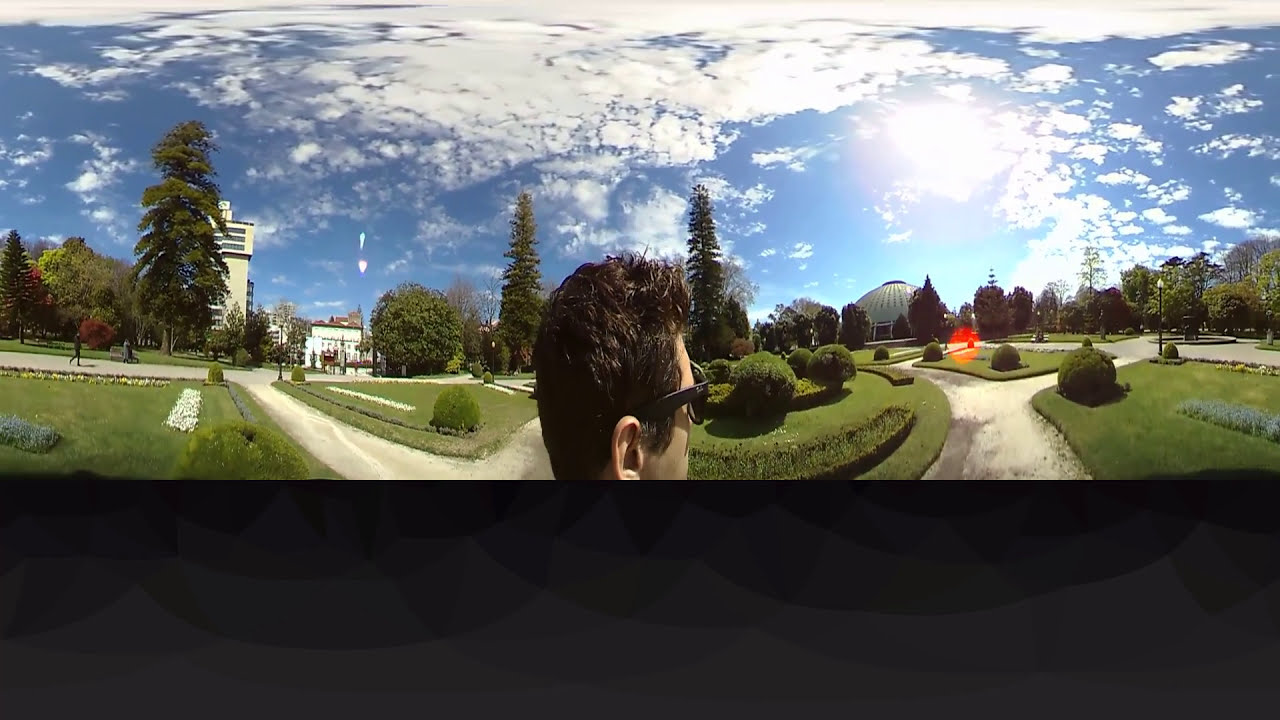In this horizontally aligned rectangular 360-degree panoramic image, we see the back of a man's head, slightly turned to the right, showcasing a bit of his profile. He sports black-rimmed sunglasses and has short brown hair styled with gel for a slightly spiked look. The man appears to be standing in a meticulously manicured garden, possibly a botanical park or a university campus. Surrounding him are manicured bushes, rounded grass areas, and intersecting beige limestone paths. To the left and right, two distinctive buildings are visible: a tall, traditional-looking building on the left and a semi-circular domed building in the distance on the right. In the near background, there's a street with pedestrians and a bicyclist making their way. The garden is dotted with both coniferous and deciduous trees, a variety of flowers, and is bathed in the light of a partly cloudy, blue sky with white feathery clouds. The image is framed by a thick black border at the bottom, adorned with subtle geometric shapes.